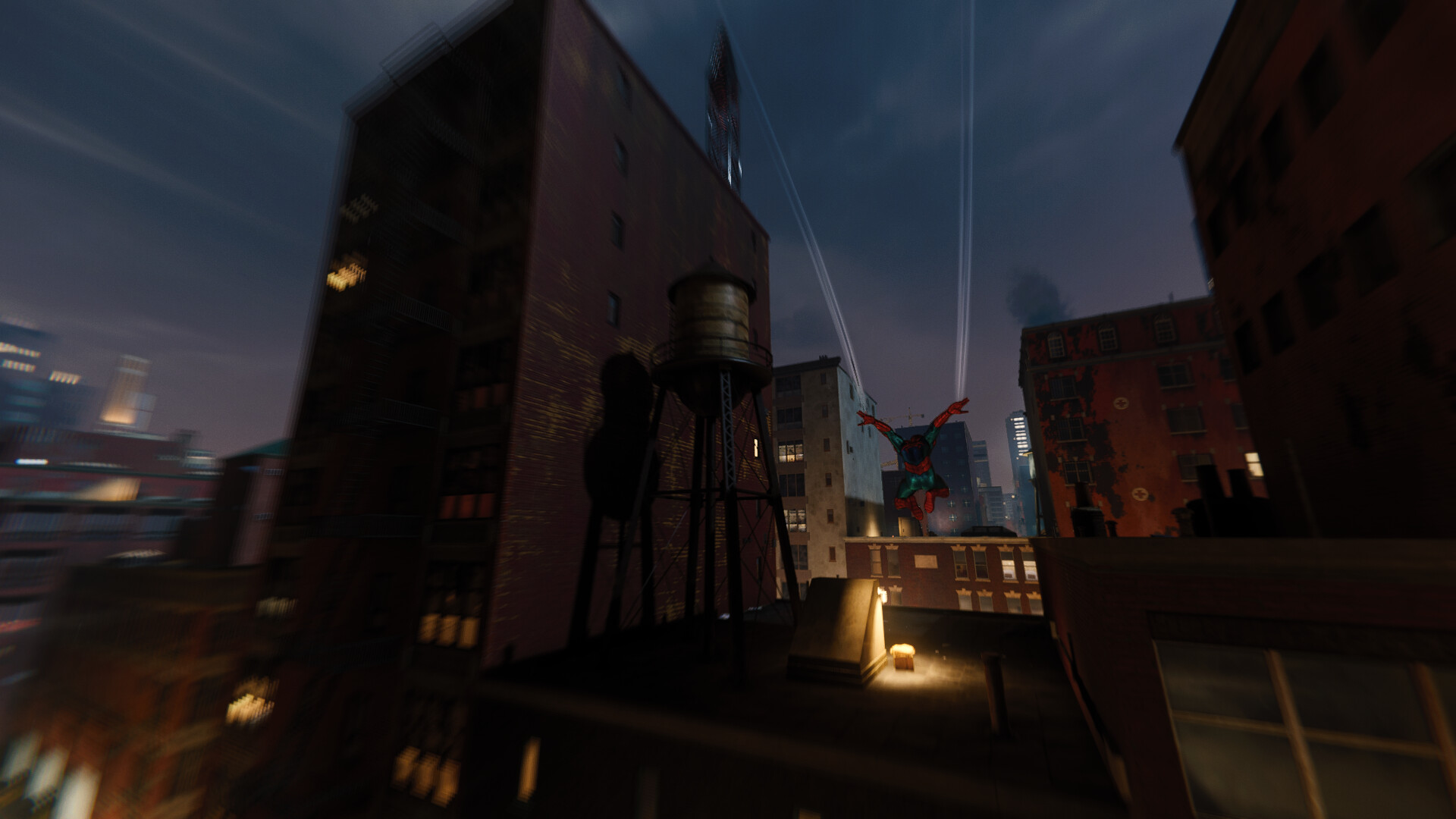The image appears to be a captivating scene from a video game set in a bustling cityscape, and it is taken at night. The sky is an enchanting shade of light mauve, interspersed with dark grey clouds, adding a dramatic flair. Central to the scene is Spider-Man, dynamically posed with webs shooting from each hand, elevated above his head as he swings through the urban jungle. On the left, a prominent large brown building stands with several windows aglow, casting warm light into the night. Atop this building is a water tower, intricately detailed, while Spider-Man sails through the air above this rooftop. To his right, a cluster of reddish-brown buildings adds depth to the cityscape; one of these structures has a single illuminated window that punctuates the darkness. In the distant background, the silhouettes of towering buildings loom, completing the rich, immersive city atmosphere.